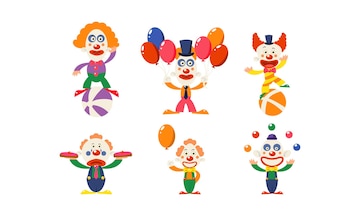The image depicts six colorful cartoon clowns against a white background, arranged in two rows of three. The clowns share similar facial features, predominantly white faces with exaggerated expressions. Starting from the top left, the first clown has vibrant orange hair, a red nose, and a broad red mouth. He wears a purple shirt with red buttons, a red bow tie, green pants, and red shoes, and is balancing on a purple and white ball. Next to him, the middle clown holds six balloons—two pink, two red, one orange, and one blue—and sports an orange shirt and pink pants. On the top right, a clown with yellow hair balances on an orange and white ball, wearing a blue top hat.

In the bottom row, the clown on the left holds two pies and dons green and blue coveralls, looking rather sad. The center clown in the bottom row holds a single orange balloon in his left hand and is dressed in matching orange coveralls. Finally, the bottom right clown, who has blue eyes, is actively juggling balls, adding to the lively scene. Each clown's distinctive attire and props create a colorful, whimsical tableau with dynamic activities.